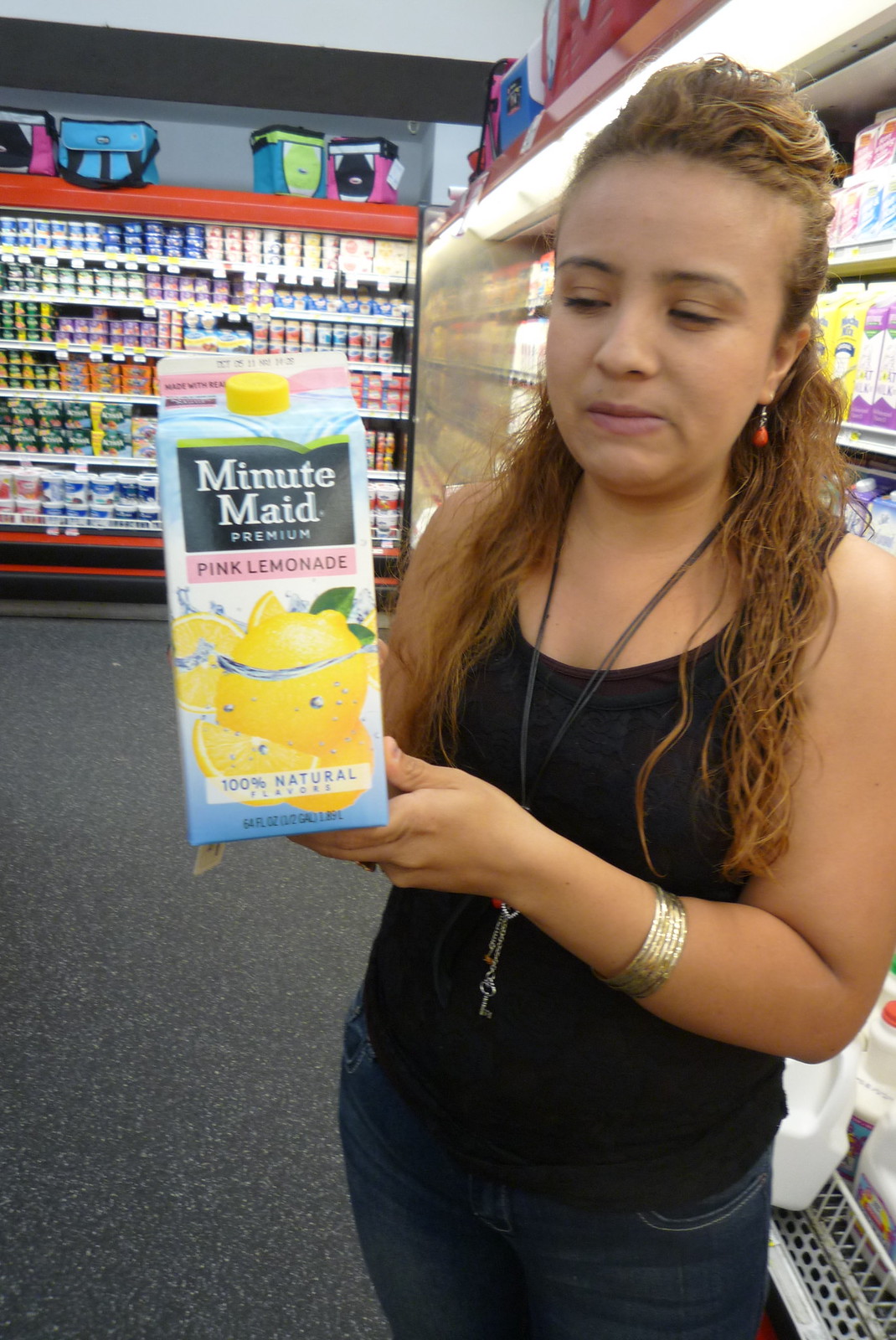In the image, a girl stands in a grocery store, holding a 64-ounce carton of Minute Maid pink lemonade. The store's gray-tiled floor contrasts with the vibrant colors of the products around her. Behind her, there is a dairy shelf topped with multi-colored coolers stocked with various items, including a selection of yogurts visible at the top part of the picture.

The girl is adorned with several accessories: she wears multiple bracelets on her arm, a black tank top, and a distinctive long black necklace featuring chains and small keys that hang around her neck. Her earrings are notable for their orange teardrop design. Her hairstyle is unique, with her hair pulled back on top and left long at the bottom, giving her a modern and stylish look.